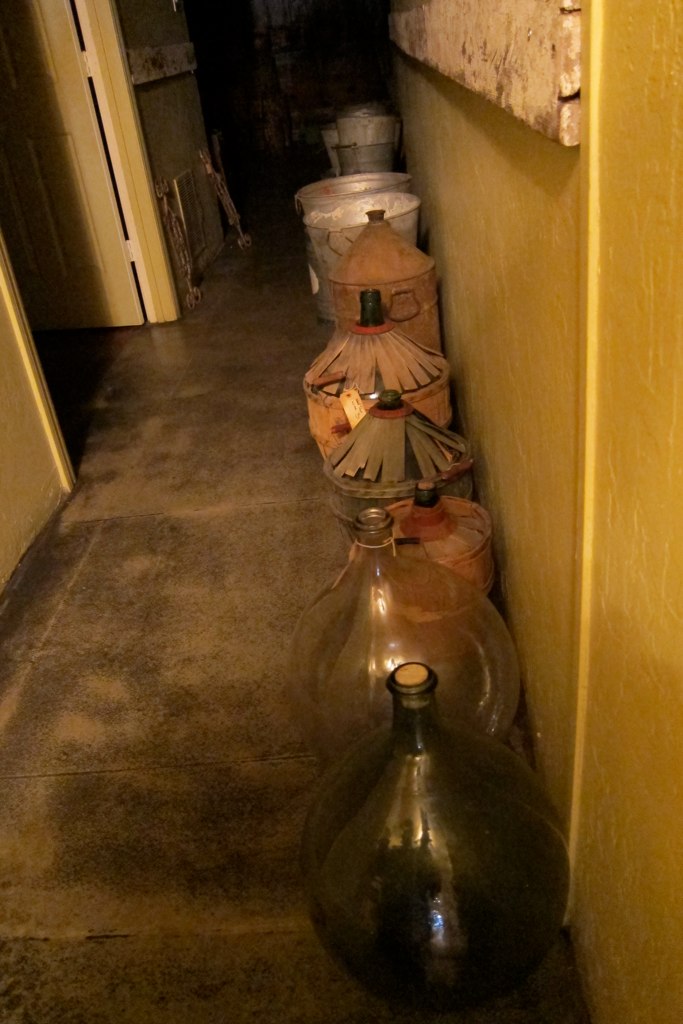The photograph captures a long hallway with light brown wood-paneled walls and a smooth concrete floor. The right side of the hallway is lined with a variety of old and used storage flasks and containers. These flasks range in material from dark tinted and clear blown glass to rusted, galvanized metal, some wrapped in protective outer coatings of woven wicker. The frontmost containers include two large round glass bottles, one clear and one green-tinted, with corks in the top. Following these are several metal canisters, one resembling a milk canister, and beyond those sit several large silver buckets. On the left side of the hallway, there is an open yellow door. Hanging on the walls are old lamps with clay bases and brown shades, along with a large piece of brown pottery. The walls and floor merge to create a scene where vintage and rustic containers reflect a sense of history and usage.